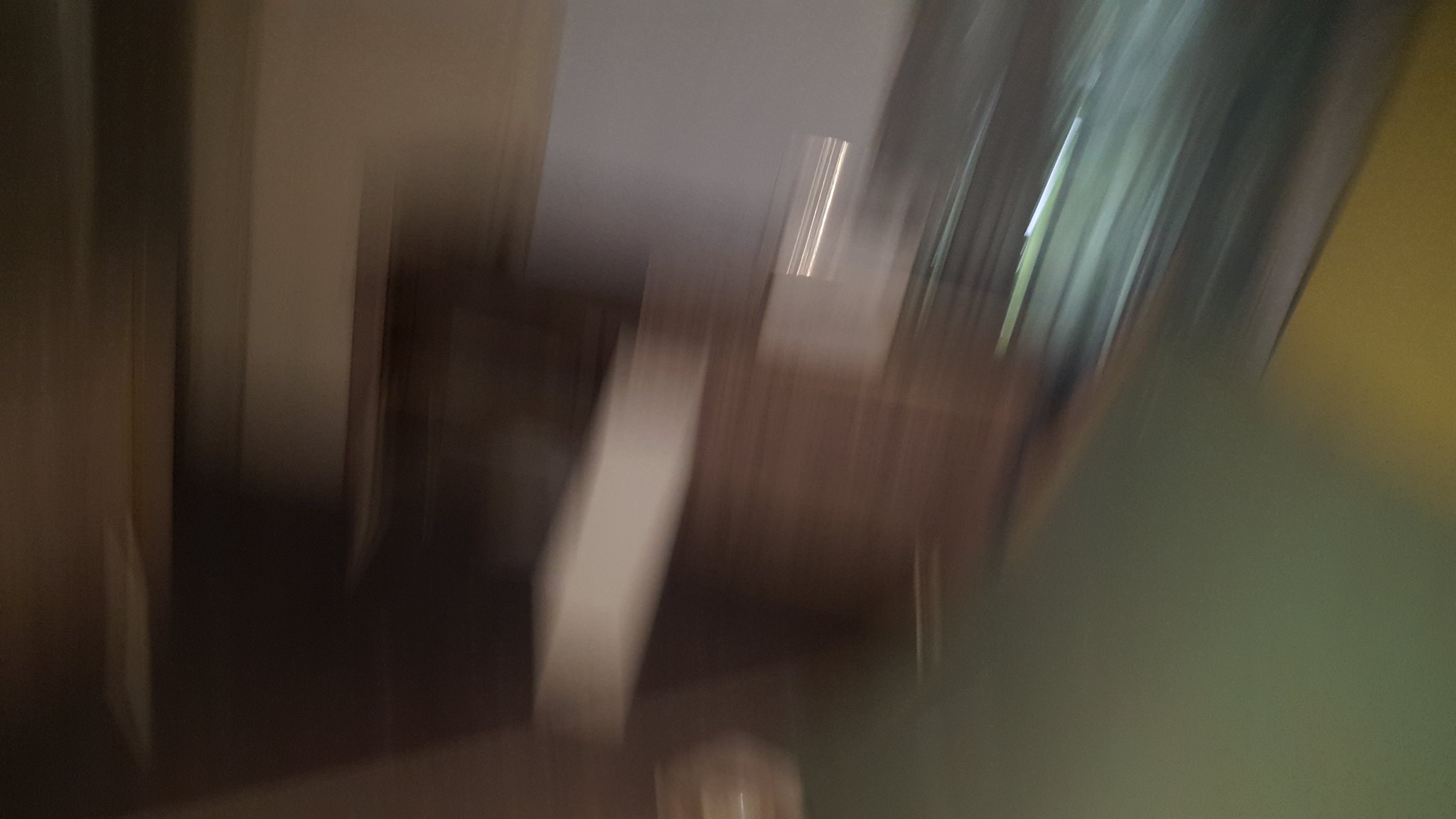This indoor photograph appears blurred due to motion during the capture. On the right side, a segment of a mustard-colored wall is visible. Adjacent to it, a doorway framed in grayish wood reveals a glimpse of some blue and white light emanating from it. Central to the image is an object that resembles a stereo or TV stand made of brown wood, topped with a white object. To the left of the stand, another doorway with a gray outline offers a view into a different room. Scattered around are several other indistinct white and brown objects, adding to the overall blurred and dynamic composition of the scene.